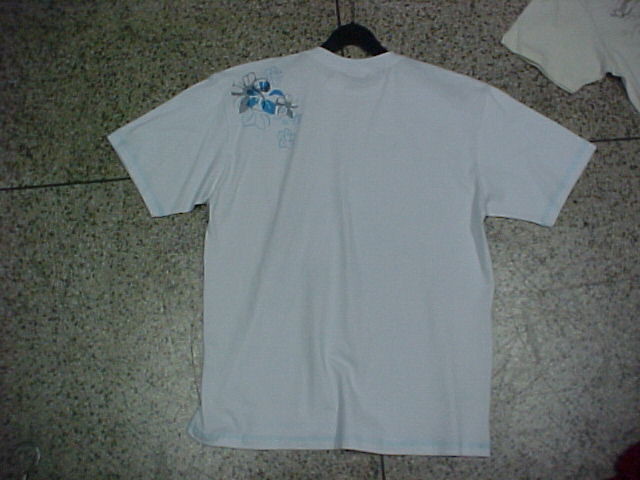The image features a tiled floor with a white, short-sleeved shirt hanging on a hanger. Positioned adjacent to it, partially visible, is another white shirt, but only one of its sleeves can be seen. The focal shirt appears to be medium-sized, likely suitable for a child. On the top left side of this shirt, there is an intricate floral design. The majority of these flowers are outlined in light blue, with four or five distinct figures. Additionally, there are two more prominent flowers in a medium to dark shade of blue. The backdrop showcases a shirt with a similar floral pattern, although this design is somewhat obscured and only parts of one flower are discernible, displaying a yellow hue instead of blue.